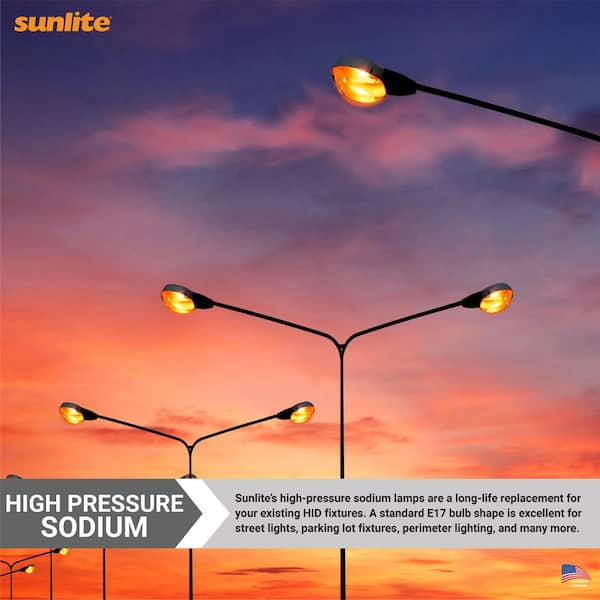The image depicts a series of black streetlights with T-shaped arms extending over both sides of a large freeway, most likely situated in the median. The lamps emit an orange glow, providing illumination as the sky transitions into dusk, featuring an orangey-red hue at the horizon that blends into a purple canopy with swirls of magenta clouds. At the top left corner, the word "Sunlight" is displayed prominently. Across the bottom of the image, an advertising panel in white font reads, "High-pressure sodium" and describes the lamps as long-life replacements for existing HID fixtures, ideal for streetlights, parking lot fixtures, perimeter lighting, and more, utilizing a standard E17 bulb shape. An American flag is discreetly positioned in the bottom right corner, suggesting that this is a promotional advertisement for Sunlight's high-pressure sodium lamps.